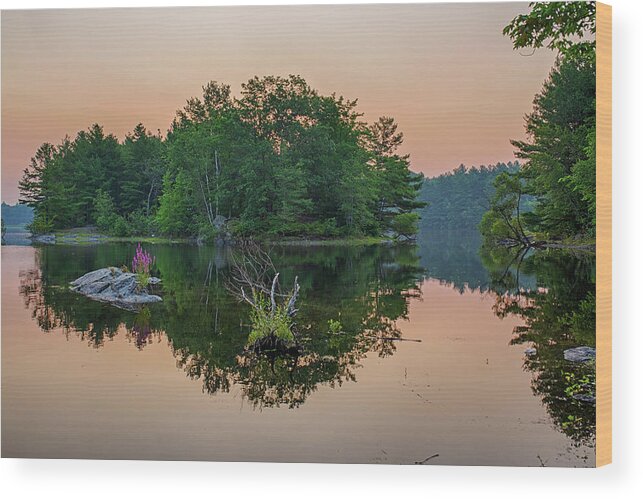This image captures the serene landscape of Pastora Lake during the tranquil moments of either sunrise or sunset. The sky is a mesmerizing blend of white at the top transitioning into a vivid orange horizon, hinting at the hidden Sun just below. At approximately a quarter mile from the left of the image, there's a picturesque island adorned with numerous deciduous trees like oak and maple, and lush vegetation. Closer to the foreground, a series of gray rocks, some decorated with delicate purple and pink flowers, lead up to a fallen, slightly rotted tree trunk sprouting grass.

To the right edge, another partially visible island peeks into the frame, featuring more trees and foliage, adding depth to the composition. In the distant background, a blurred tree line marks the mainland, effectively creating a stunning backdrop. The lake itself is astonishingly calm, with a mirror-like surface that flawlessly reflects the sky's hues and the island's form, presenting an almost surreal, artistic quality. Every element in this image, from the pristine reflections to the stillness of the water, exudes an overwhelming sense of peace and serenity.